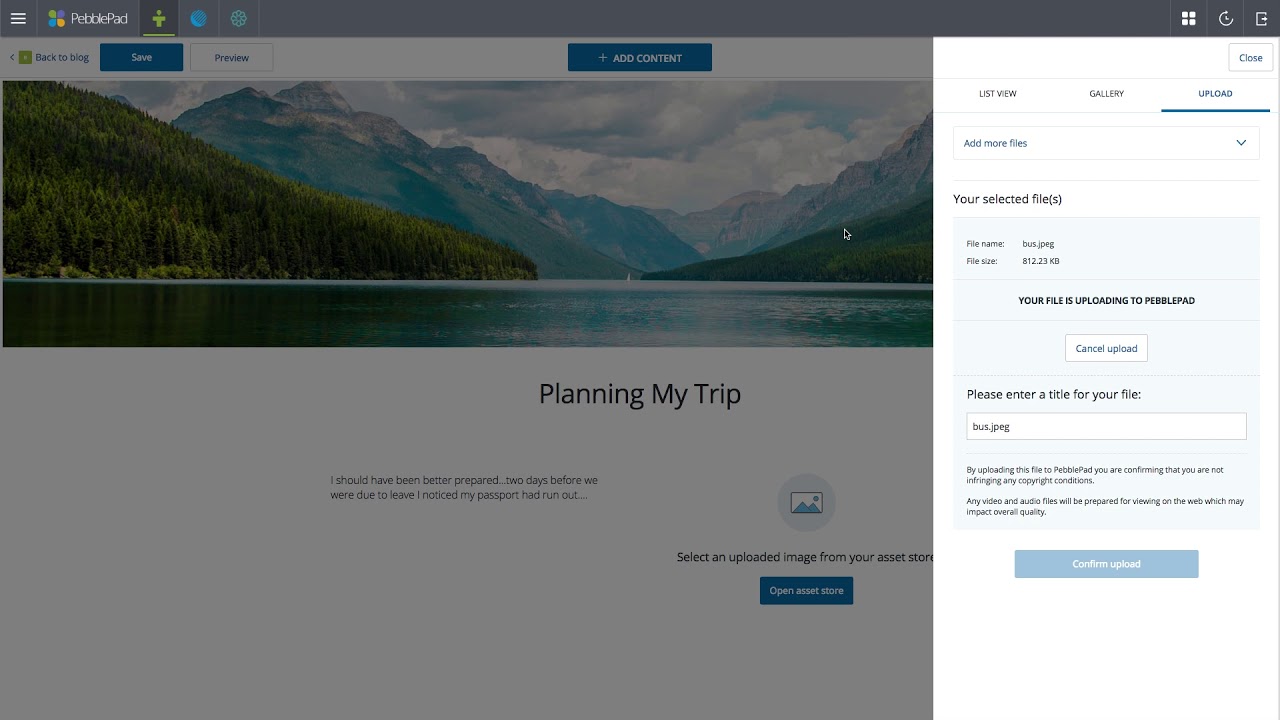The rectangular image captures a screenshot from a computer, where an individual appears to be planning a trip on a website interface. The layout is predominantly horizontal, with the longer side extending from left to right. 

At the top left, within a gray banner running along the upper edge of the screen, there are several user interface elements: a hamburger menu icon, the label "Pebble Pad" accompanied by a small figure icon, and two circles. On the right side of this banner, Windows-specific icons are visible, including a Windows logo, a clock, and a square symbol.

The bottom two-thirds of the image features a section predominantly on the left, showcasing a picturesque scene of mountains, a forest, and a lake, slightly obscured with a gray overlay. Over this image, in black text, a personal anecdote reads, "Planning my trip, I should have been better prepared. Two days before we were due to leave, I noticed my passport had run out." Below this text, instructions prompt the user to "Select an uploaded image from your asset store" or "Open asset storage."

The remaining right-hand side of the screen is a contrasting white section, seemingly designated for inputting or managing trip details, offering a structured space for planning.